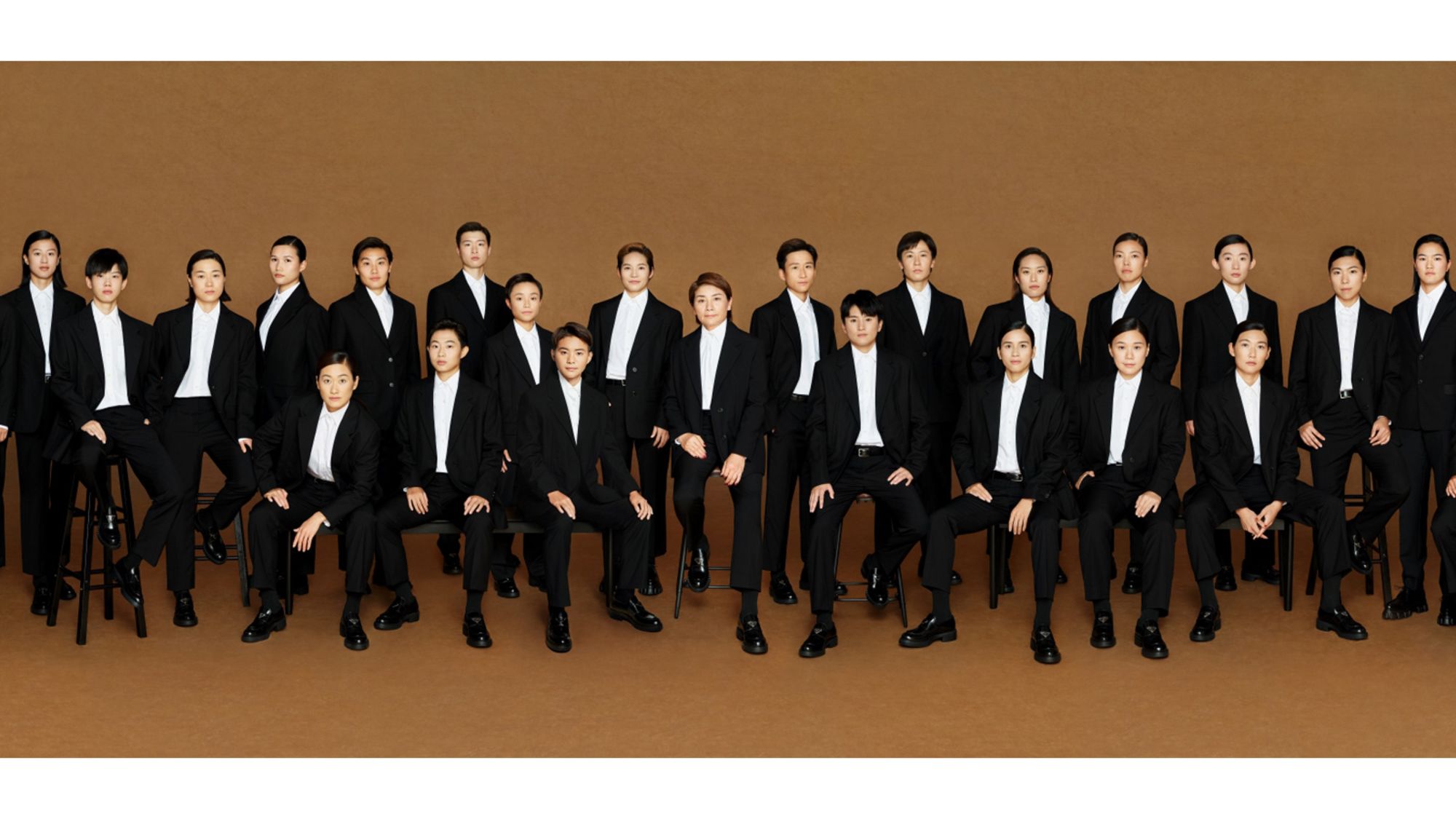The photograph captures a large group of approximately 20 to 23 people, both men and women, set against a brown background with a brown floor, giving the image a uniform and somewhat surreal appearance. All individuals are attired uniformly in black suits, consisting of black pants, black shoes, a black suit coat, and a white inside shirt. The arrangement shows the women and men posing with some sitting in black chairs or on stools in the front, while others stand in the back. Notably, the person on the far left is a woman standing and looking straight forward. The image gives the impression of a formal, possibly orchestrated group photo, with everyone looking directly at the camera.